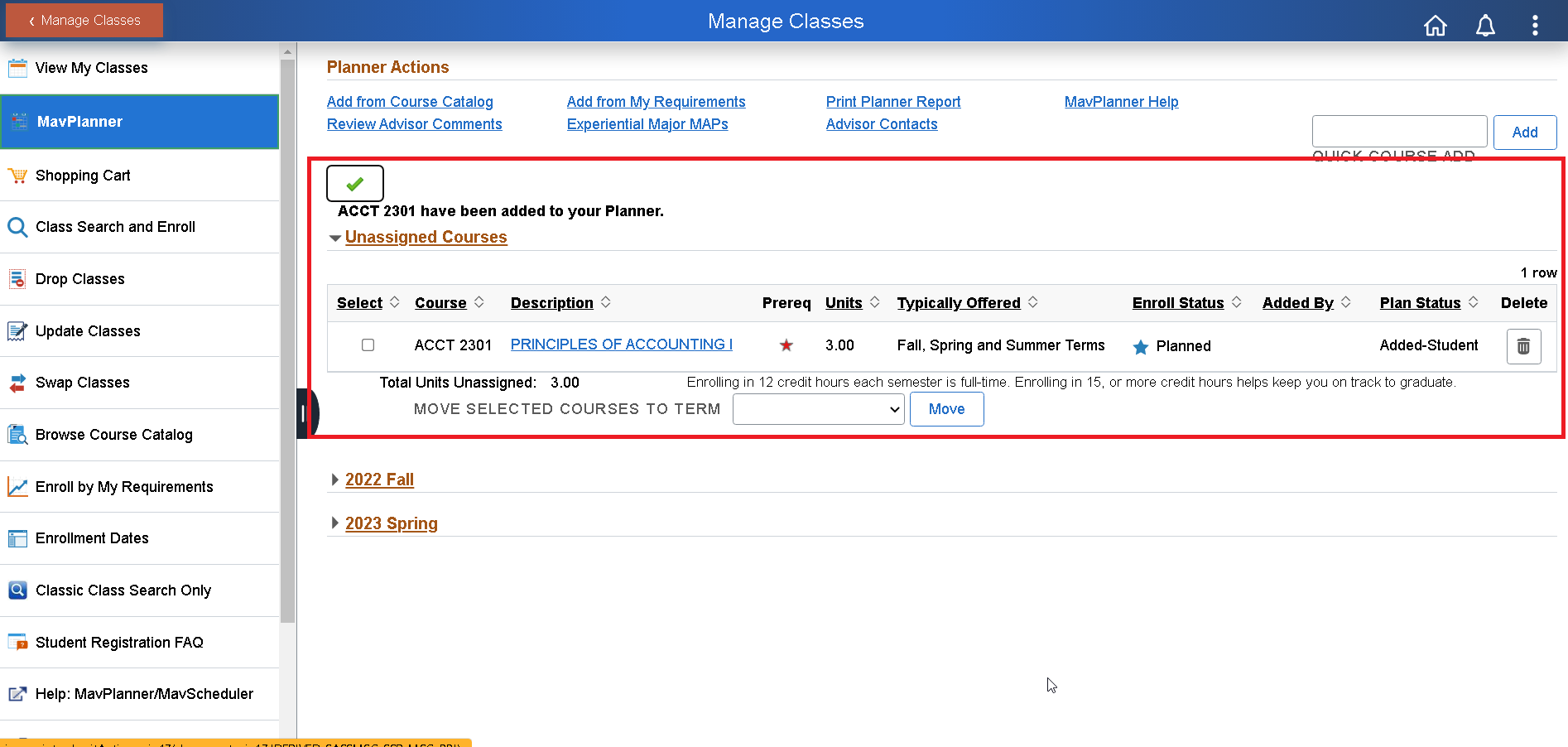This is a screenshot of a website interface dedicated to managing classes. At the upper left corner of the page, there is an orange button labeled "Manage Classes" accompanied by a left-pointing back arrow. Centrally positioned at the top is a prominent blue bar with the text "Manage Classes" displayed in white.

On the left side of the screen, a vertical navigation menu is present. It includes options such as Home, Alerts, and a three-dot Menu button. Below these primary options, the menu continues with several links stacked vertically: 
- View My Classes
- Map Planner (highlighted)
- Shopping Cart
- Class Search and Enroll 
- Drop Classes 
- Update Classes 
- Flop Classes
- Browse Course Catalog 
- Enroll By My Requirements
- Enroll Dates
- Classic Class Search Only 
- Student Registration 
- Frequently Asked Questions 
- Help: Map Planner/Map Scheduler

To the right of this navigation menu, inside the Map Planner section, there is a list of Planner Actions, which includes:
- Add From Course Catalog (Hyperlink)
- Review Advisor Comments (Hyperlink)
- Add From My Requirements 
- Experiential Major MIPs (Hyperlink)
- Print Planner Report (Hyperlink)
- Advisor Contacts (Hyperlink)